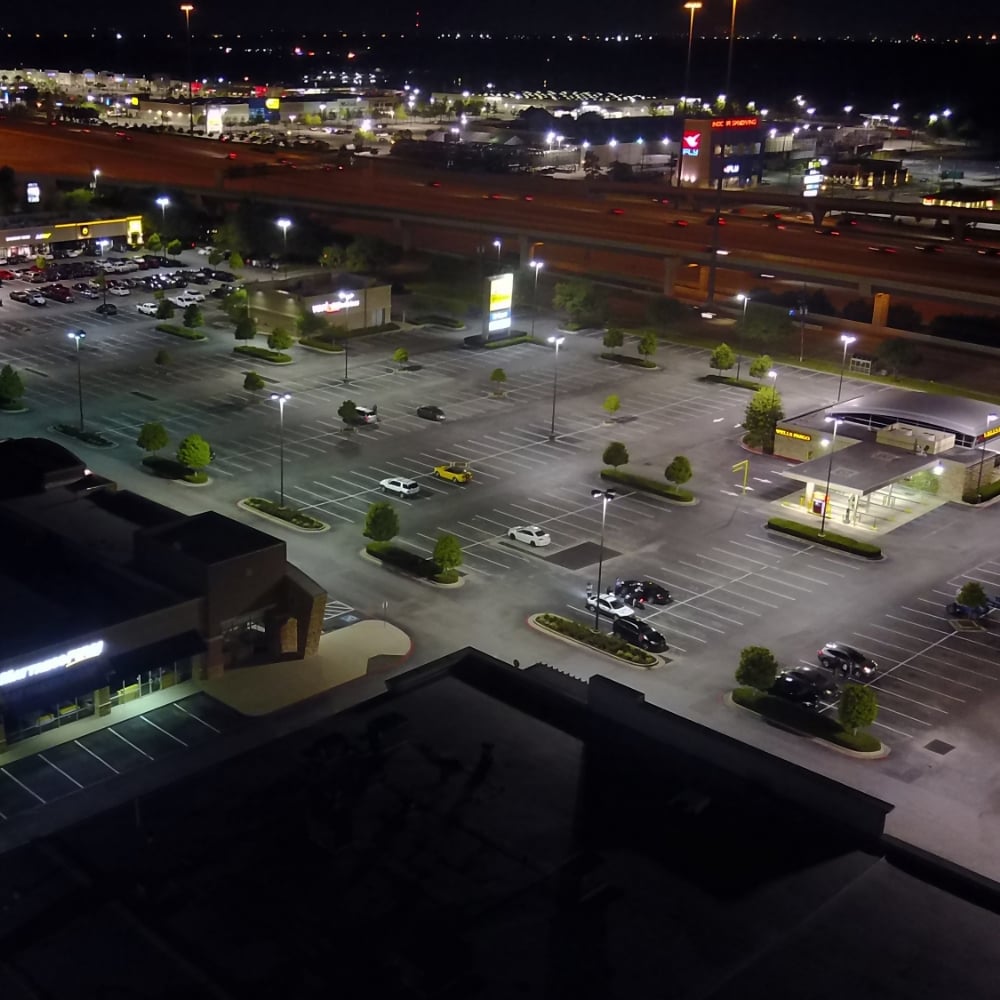The aerial nighttime photograph captures a sprawling outdoor mall parking lot, illuminated by ambient lights from surrounding buildings and streetlights. The dark sky above emphasizes the well-lit area below, highlighting the intricate layout of roads leading into and out of the expansive parking spaces. Prominently visible is a building with a glowing blue sign that reads "FLY," possibly a commercial or retail store. Additionally, a Wells Fargo branch is identifiable by its distinctive yellow and red signage, complete with an ATM. Scattered throughout the parking lot are various vehicles in a range of colors, including black, silver, yellow, and white, adding to the scene’s vivid detail. The image provides a comprehensive view of a bustling nighttime commercial area, blending the stillness of night with the activity of late-hour shoppers and commuters.